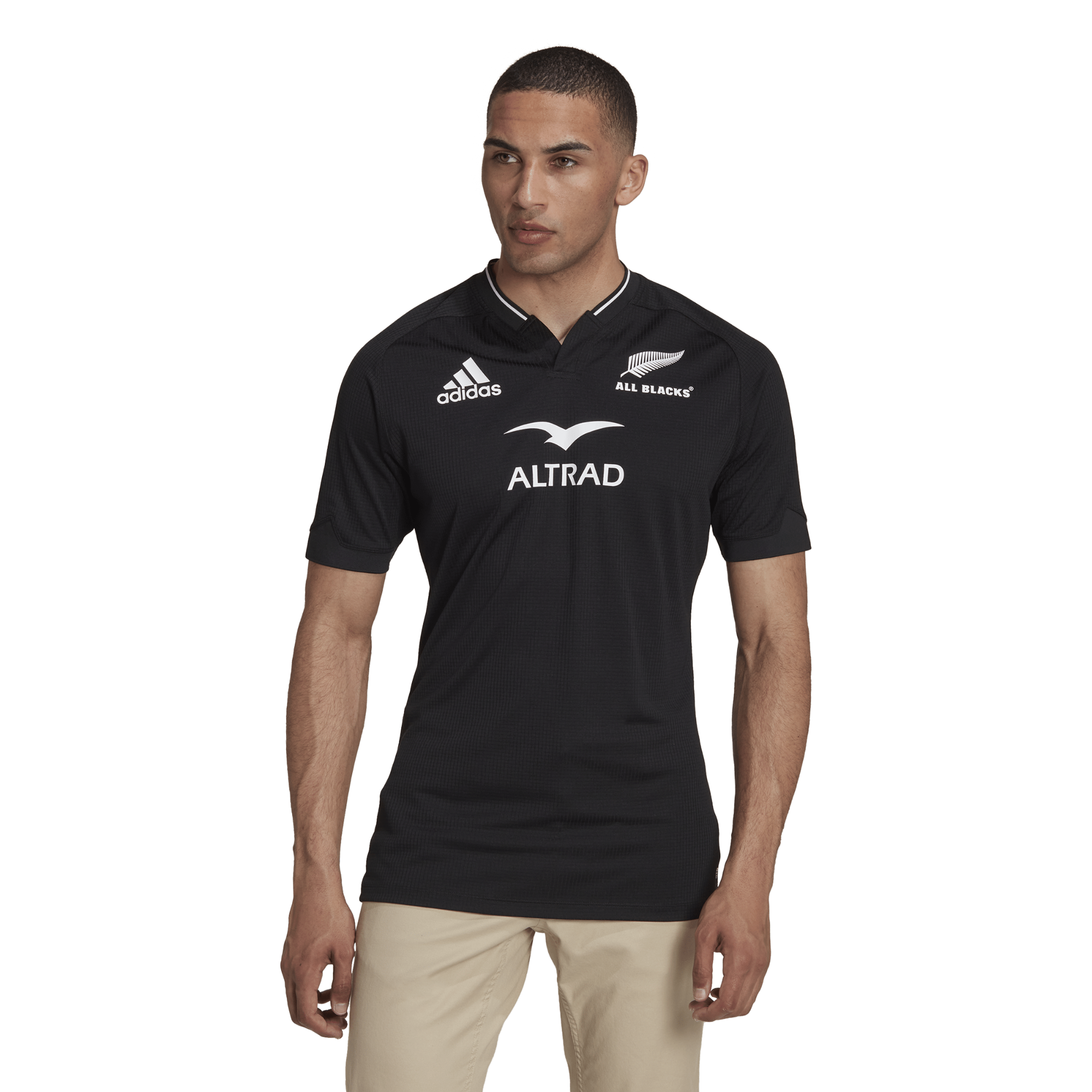The image shows a man modeling clothes, standing against a plain white background. He is wearing a black Adidas jersey with the Adidas logo on the upper left side and the word "Altrad" along with a white bird symbol on the upper right. The shirt also features the words "All Blacks" alongside a feather. His shirt has short sleeves and a collar with a white stripe around it. The man is dressed in tan khaki pants and has a thin, muscular build with visible veins on his forearms. He has a short buzz cut and light brown skin with clearly defined features, including big lips, tall eyebrows, a straight nose, a chilled jawline, and brown eyes. His nails are trimmed, and both hands are slightly curled at his sides. The man is looking off to the left, with a focused expression and legs slightly parted. He wears no jewelry.